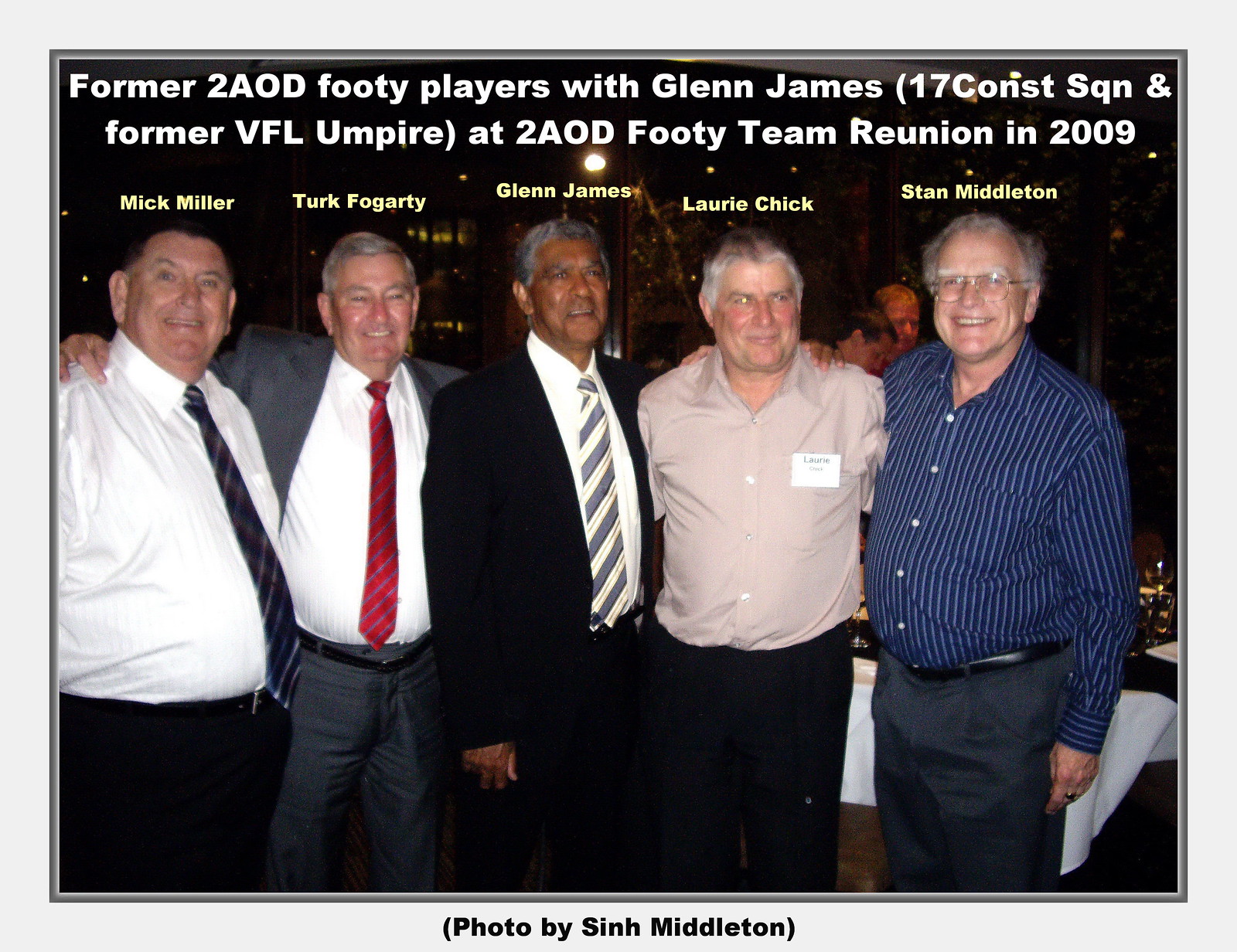The photograph captures a close-up of five middle-aged to older men, dressed in business attire, standing shoulder-to-shoulder with their arms draped over one another’s shoulders. They are all smiling and looking directly at the camera. The men are positioned from left to right as follows: Mick Miller, Turk Fogarty, Glenn James, Lori Chick, and Stan Middleton. Four of the men are white, while the third man, Glenn James, appears to be either Black or Indian. The photograph features a blue border and a yellow watermark above each man's head indicating their name in yellow text. At the top of the image, a white caption reads: "Former 2AOD footie players with Glenn James (17 Const SQN and former VFL umpire) at 2AOD footie team reunion in 2009." The man on the far left is dressed in a shirt and tie, the one next to him has a jacket and tie, followed by another in a jacket and tie, then one in a shirt and dark pants, and finally, the man on the far right is in a striped shirt and dark pants. At the bottom of the image, it states "photo by Sinh Middleton."